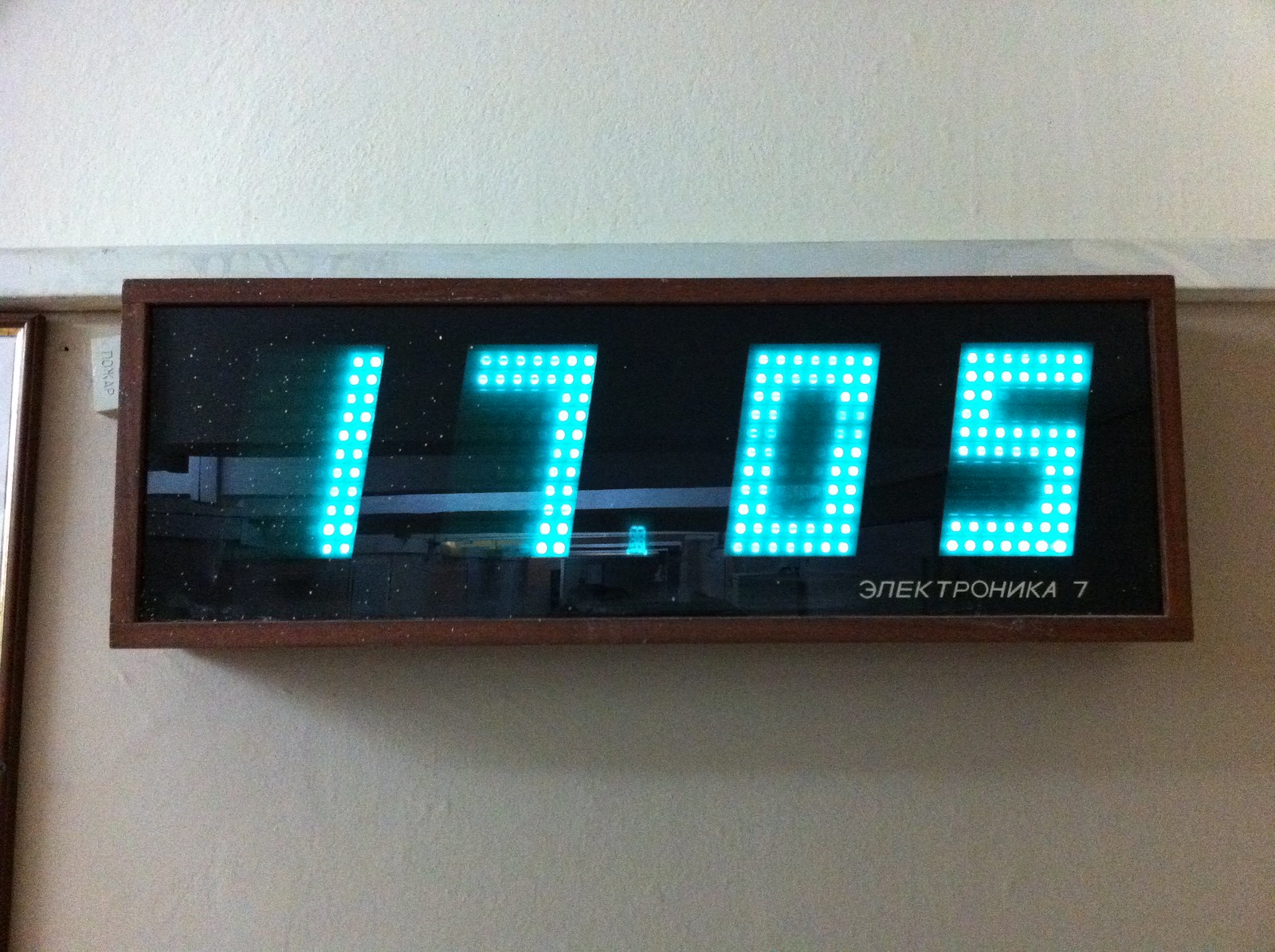This horizontally-oriented color photograph features a prominent wall-mounted clock. The clock, which is presumed to be large, has a brown border framing a black digital display. The display screen showcases the numbers "17:05," slightly tilted to the right, in block letter format. These numbers appear to be illuminated with white lights, set against a blue background made up of several lit dots. Beneath the number "05," there is some white text, presumably in Russian, suggesting that this could be a countdown timer, possibly used during a sports event. The clock is mounted on a beige wall with a decorative border above. The upper part of the wall transitions into a white stucco surface, adding a contrast between the textures.